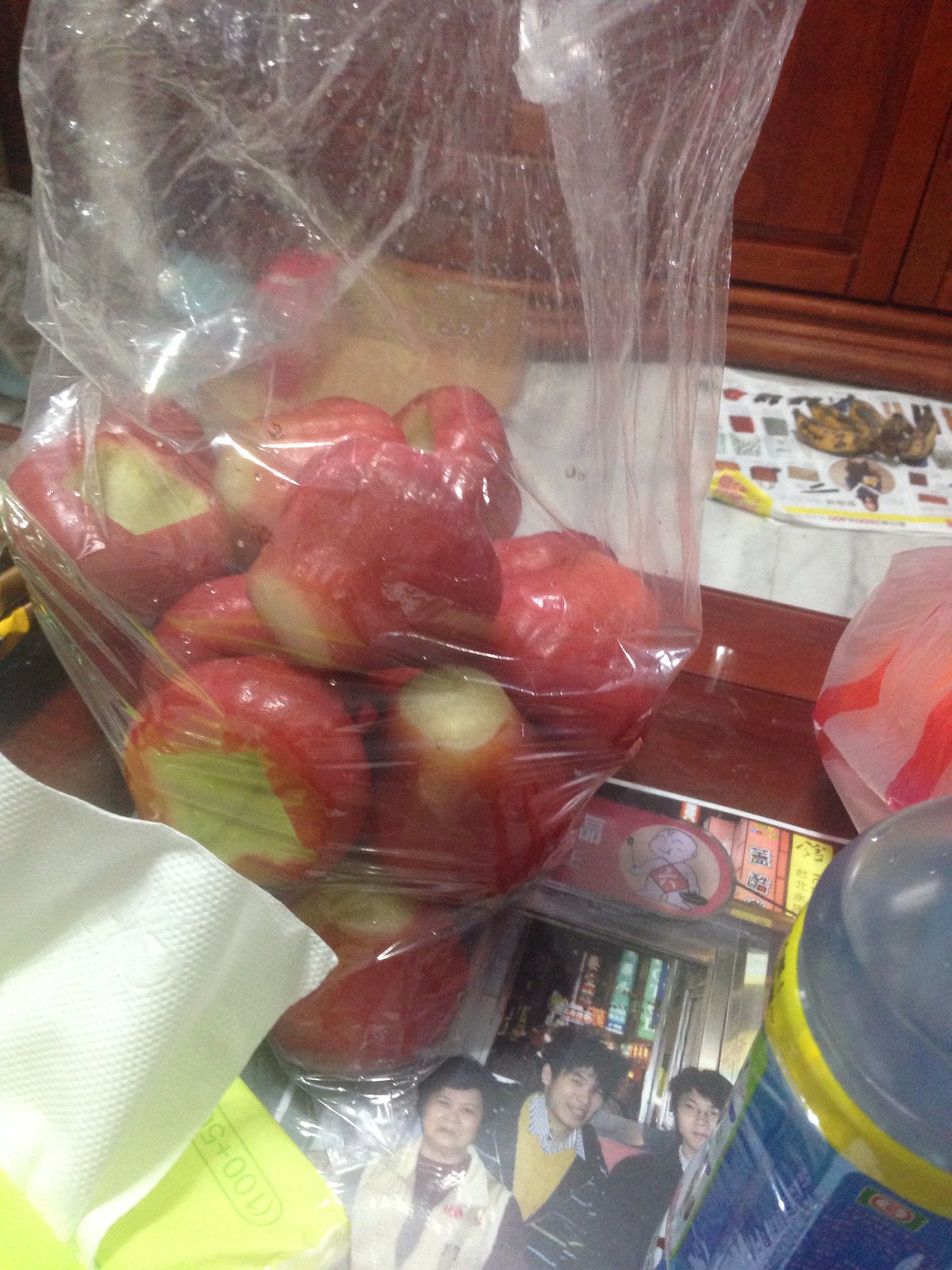In this image, the central focus is a clear plastic bag filled with small, reddish fruits that appear to be apples, though they might also be radishes or onions. The bag is placed on a wooden coffee table. Surrounding the bag are several objects: a partial box of Kleenex with white tissues sticking out, an olive green box with some text, and a water bottle with a yellow and blue label. At the bottom center of the image, there is a family photo featuring a Japanese woman and two boys. The background features maroon or reddish-brown cabinets and a white mat. Additionally, there are water droplets visible inside the bag, and a shrimp on a paper is also faintly visible at the back of the table. The scene is well-lit, highlighting the various elements on the table.